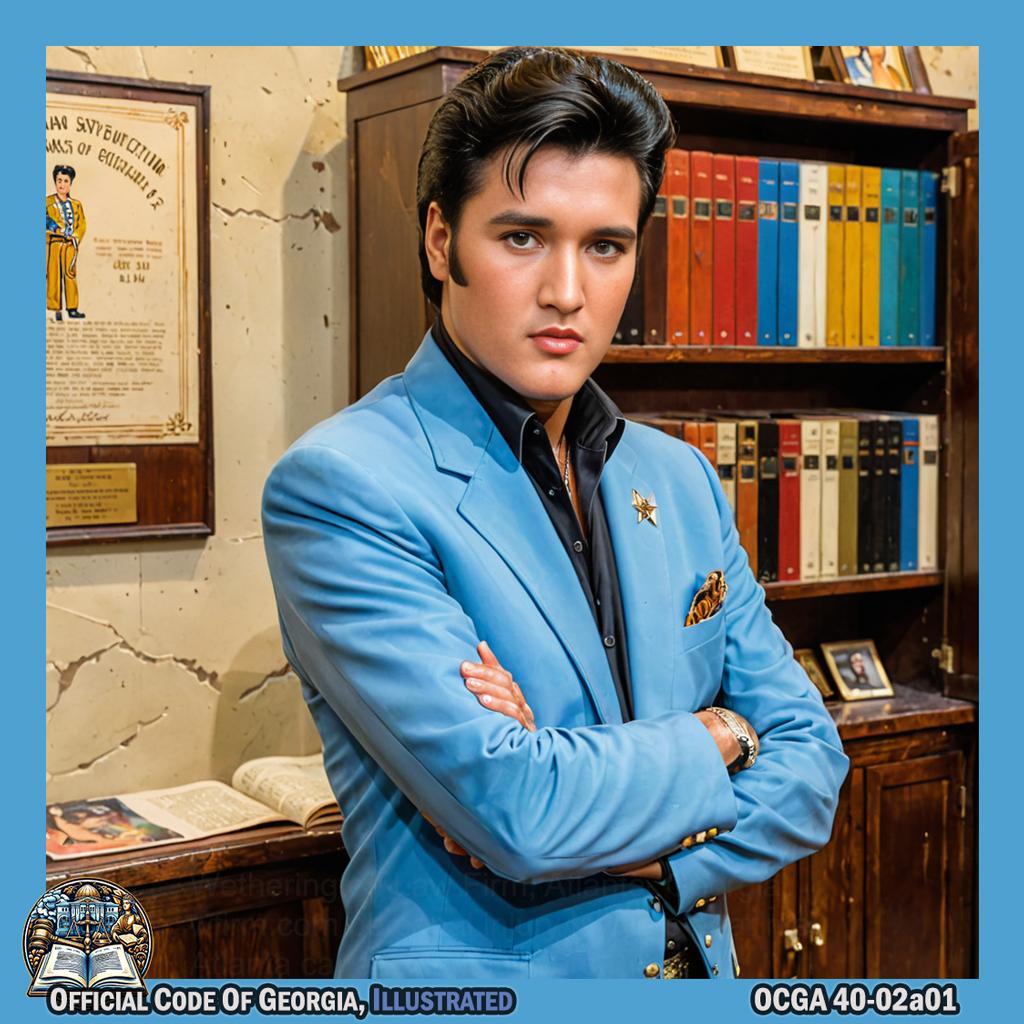The image depicts a young Elvis Presley, or someone who closely resembles him, standing confidently with his arms crossed and his body slightly turned to the right. He is attired in a powder blue suit jacket adorned with gold buttons, a gold star, and a gold kerchief in the breast pocket, over a black button-down shirt. The portrait-style artwork is enclosed in a blue border, with the inscription "Official Code of Georgia, Illustrated" at the bottom in light gray, alongside the identifier "OCGA40-02A01".

In the background, a wooden bookshelf is visible, filled with variously colored books—arranged in an orderly fashion on the top shelf with colors ranging from blue, yellow, and white to red, orange, and brown. The second shelf features a more mixed arrangement of blue, white, black, and red books. Additionally, a framed award hangs on the wall next to the bookshelf, which itself appears somewhat cracked, adding a touch of antiquity to the scene.